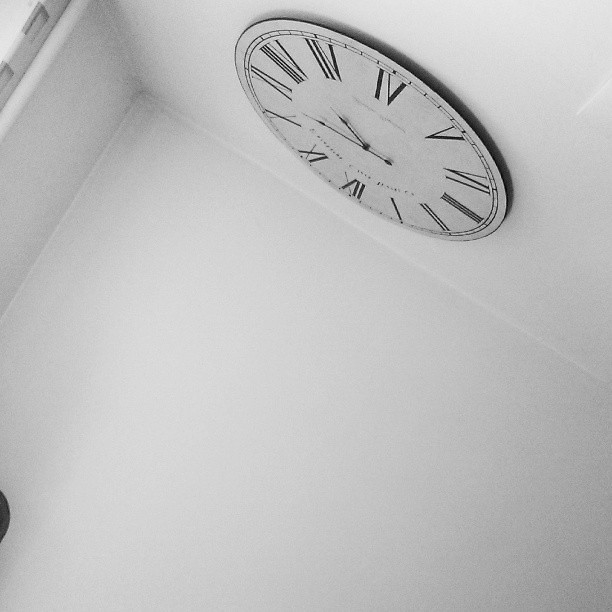In this image, we see a classic wall clock featuring black Roman numerals on a white face, framed by black trim. The clock, which displays the numbers 12 and 6 prominently flanking the top, appears to hang near the corner of a white room, as it is viewed from an unusual upward angle. This perspective makes it look almost as if the photographer is upside down. The hands of the clock are also black, and there is some writing near the 12, though its content is unclear. The clock is mounted on a white wall close to the corner where the ceiling, also white, meets another white side wall. In the upper left corner, there appears to be a window, and at the bottom left of the image, a small black half-circle can be seen entering the frame.